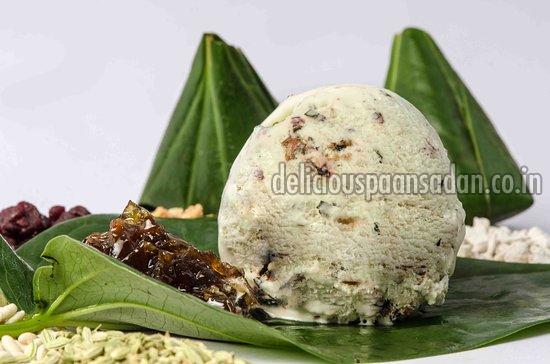The photo features a high-end dessert elegantly presented on a large, dark green banana leaf. At the center of this presentation is a nearly perfect scoop of white ice cream, speckled with small brown and black bits that suggest the inclusion of fruits or nuts, possibly dates and raisins. To the left of the ice cream, there is a thick, viscous syrup or sauce with a rich, honey-like appearance and texture akin to jelly or toffee. Surrounding the main components, the background showcases two cone-shaped, leaf-wrapped parcels, adding a decorative touch and possibly indicating how the dessert is served. Additional details include a mix of nuts or grains at the bottom of the image and a credited website at the top stating 'deliciouspansadan.co.in.'